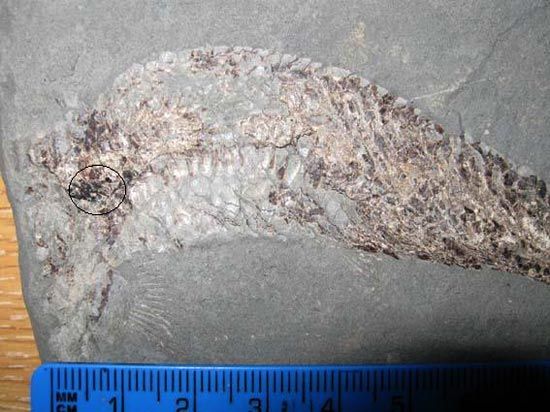This image showcases a detailed close-up of a fossil embedded in a large gray rock, which rests on a wooden surface. The fossil, resembling the shape of a fish or possibly a serpent, exhibits discernible bones and what appear to be scales, all in varying shades of gray, dark red, black, and brown. One noteworthy detail within the shape is a distinct, very small circle outlined in black, located on one of the darker segments of the fossil. The texture of the fossil contrasts with the surrounding stone, appearing jagged and rough. At the bottom of the image, a blue ruler marked in millimeters and centimeters extends across the scene, measuring the fossil's length. The ruler, visible up to the fifth centimeter, is partially obscured by a dark shadow on the right side, making it difficult to determine the fossil's full length.